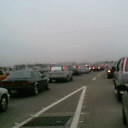This image, taken from within a car in a traffic jam, captures a congested road scene. At the center of the image is a white line that extends upward one third of the way, creating an upside-down V shape before slanting leftwards. Beneath this white line, a large black grate contrasts against the surrounding lighter gray pavement. On the right side, several cars are visible, including a silver vehicle with illuminated taillights. The left side features a snippet of a silver car's front bumper, followed by a black car, then another silver one, as the vehicles blur into indistinctness in the distance. Taillights punctuate the scene with occasional red glows. The road, in good condition, is gray and stretches far into the backdrop where a subtle tree line is just discernible. Across the top half of the image, patches of a blue sky peek through the otherwise gray, overcast atmosphere, lending a dreary tone to the overall scene.